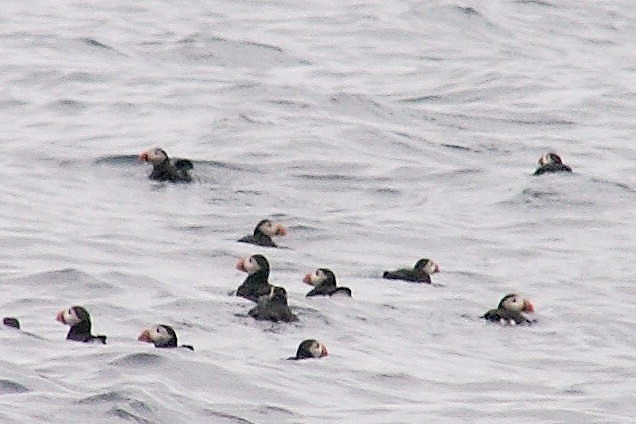The image depicts a large group of puffins leisurely swimming in choppy, dark gray waters that range from shades of dark to light gray. These seabirds are characterized by their distinct appearance: they boast black bodies, white faces, and prominent orange beaks. The puffins are scattered across the scene, with about ten visible in the foreground and a couple more in the distant background. The water they are floating in has a visibly wavy and somewhat turbulent surface, creating ripples that partially obscure the puffins, especially towards the bottom left of the image. The photograph has a grainy texture, which reduces the overall detail, but it still captures the serene yet dynamic nature of the puffins amidst the swirling water.